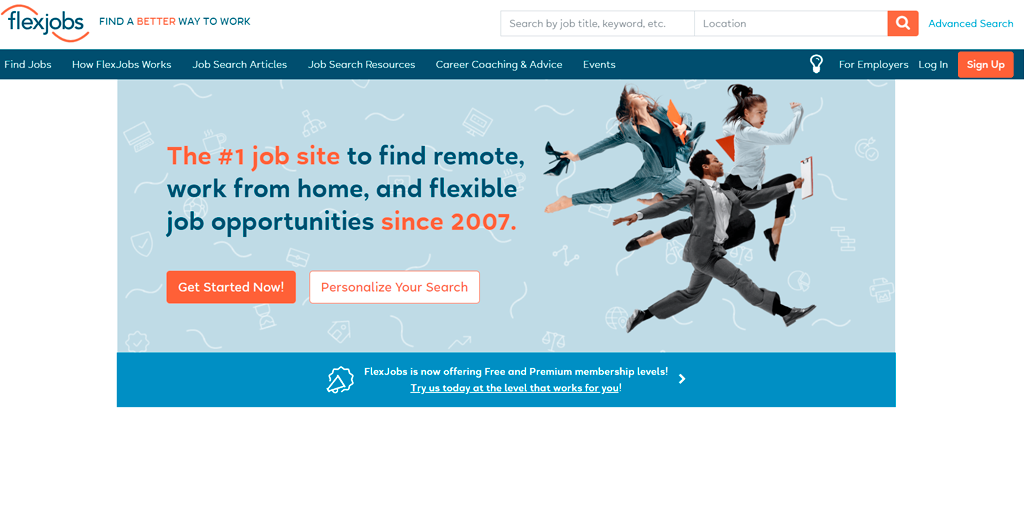This image captures the homepage of the FlexJobs website. At the top center, the FlexJobs logo is prominently displayed, accompanied by the slogan "Find a better way to work" in vibrant blue and orange colors. Below the logo, a search bar is visible, allowing users to look for jobs by title, keyword, or location, complete with a white magnifying glass icon on an orange background. To the right of the search bar, there is an option for an advanced search, highlighted in blue. 

The navigation menu includes various categories such as "Find Jobs," "How FlexJobs Works," "Job Search Articles," "Job Search Resources," "Career Coaching & Advice," and "Events." Along the top right, there are buttons for "For Employees," "For Employers," a login button, and an orange 'Sign Up' button.

Dominating the central part of the image, a bold headline states, "The #1 Job Site to Find Remote, Work from Home, and Flexible Job Opportunities Since 2007." Beneath this proclamation, an orange "Get Started Now" button and a "Personalize Your Search" option in white invite users to take action. 

The image also showcases an energetic array of people dressed in professional attire, joyfully jumping in the air, symbolizing the excitement of finding flexible job opportunities. 

At the bottom, an announcement on a blue background states, "FlexJobs is now offering free and premium membership levels. Try us today at the level that works for you." The majority of the page has a clean white backdrop, while the top section features a darker blue background.